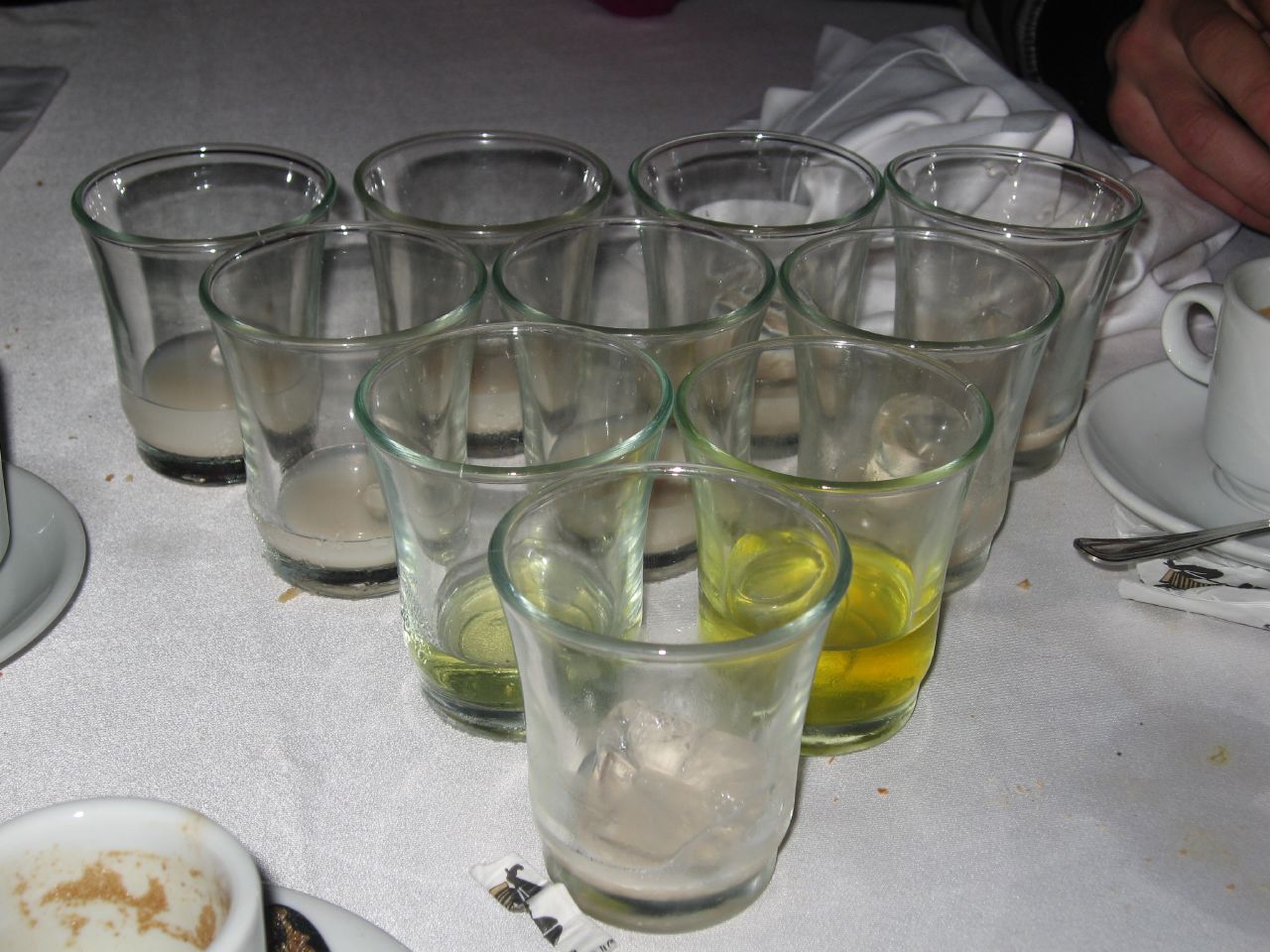The image showcases a table adorned with a pristine white tablecloth, centrally featuring ten short, clear glass shot glasses arranged in a pyramid formation: a back row of four, then a row of three, followed by a row of two, and finally a single glass at the front. Some glasses contain varying amounts of liquid, with light brown liquid in the front glass and several in the back row. The second row includes one glass with a clear liquid and another with a yellow beverage, suggestive of a beer-like substance. A white ceramic bowl with remnants of brown food sits towards the bottom left, and a torn wrapper is placed near the foremost glass. On the middle right, there is a white ceramic teacup on a matching saucer, accompanied by a silver teaspoon, and a white cloth napkin is located next to the back row of glasses.